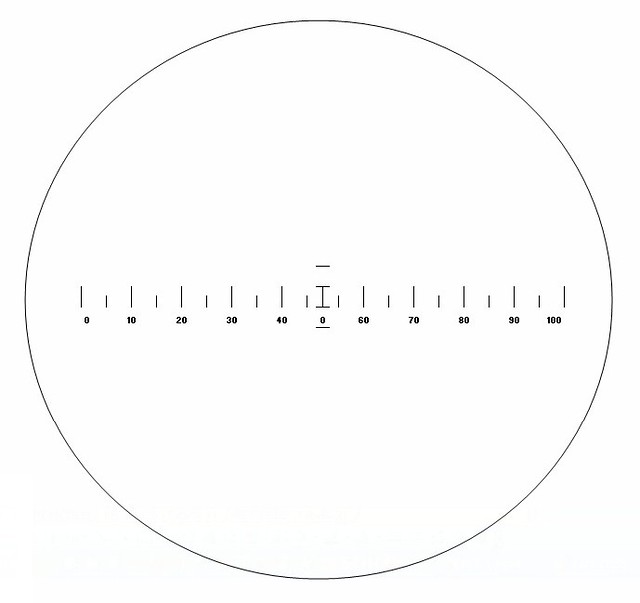The image displays a simple, circular scope-like graph on a white background. The circle is outlined in light black or gray. Along the horizontal diameter of the circle, there are numbered measurements from 0 to 100 in intervals of 10, with each number corresponding to a longer vertical dash and shorter dashes in between for finer divisions. The numbers start from 0 on the left side, progressing through 10, 20, 30, and up to 40 in the center. The central section features an emphasized 0, flanked by two dashes on each side, underneath an eye-shaped figure, which is aligned with a horizontal line crossing the circle. The sequence continues from 60, 70, 80, 90, and finally to 100 on the far right. All lines are aligned vertically below their respective numbers except for the central horizontal line. The overall presentation suggests a measuring or focusing instrument with its evenly spaced numerical scale.